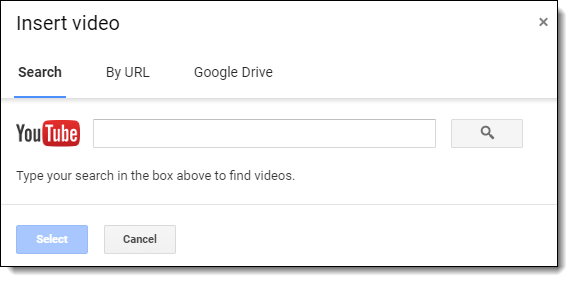This screenshot depicts a YouTube dialog box for video insertion, emphasizing the search functionality. At the top left corner of the rectangular dialog box, the label "Insert Video" is prominently displayed. Directly below this title is the search options menu, which offers three selectable links: "Search" located centrally, "By URL" positioned to its right, and "Google Drive" on the far right. Beneath these options, the familiar YouTube logo is situated, signifying the search context. To the right of the logo rests an elongated rectangular search bar, accompanied by a microscope icon—denoting advanced search or scrutiny—towards its right end.

Further down, black text on a white background directs the user with the instruction "Type your search in the box above to find videos." At the very bottom of the dialog box, two buttons are aligned horizontally in the bottom left corner. The first button, light blue with white text, reads "Select," while the adjacent grey button, featuring black text, provides a "Cancel" option. This detailed interface layout is designed to facilitate efficient video searches and selection within the YouTube ecosystem.